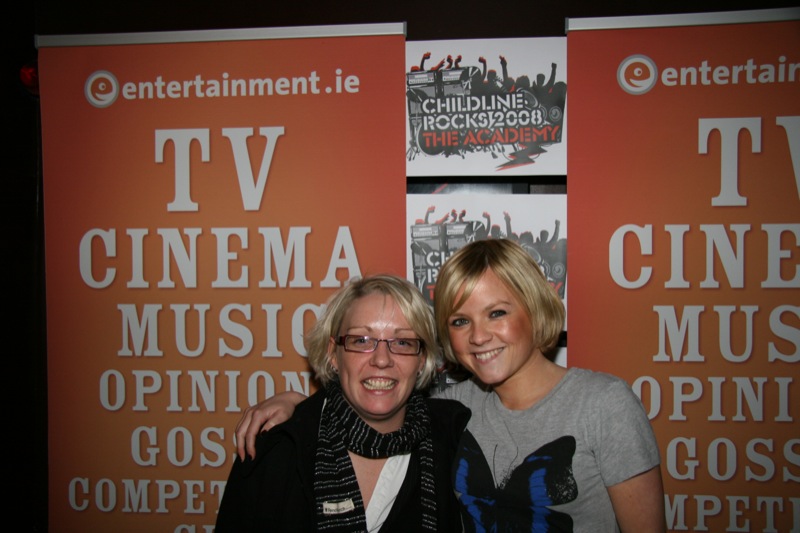Two blonde women, an older woman on the left and a younger woman on the right, are posing and smiling in front of two identical orange promotional banners with a silver frame. The banners prominently feature white uppercase text that reads "entertainment.ie, TV, Cinema, Music, Opinion, Gossip, Competition." Between the larger banners are smaller square-shaped signs that announce "Childline Rocks 2008, The Academy." The older woman on the left is wearing brown-rimmed glasses, a black sweater, and a black and white striped scarf, while the younger woman on the right sports a gray short-sleeve graphic T-shirt adorned with an image of a black and blue butterfly. Both are positioned against a dark backdrop that contrasts with the vibrant orange of the promotional banners, emphasizing the event's celebratory atmosphere.